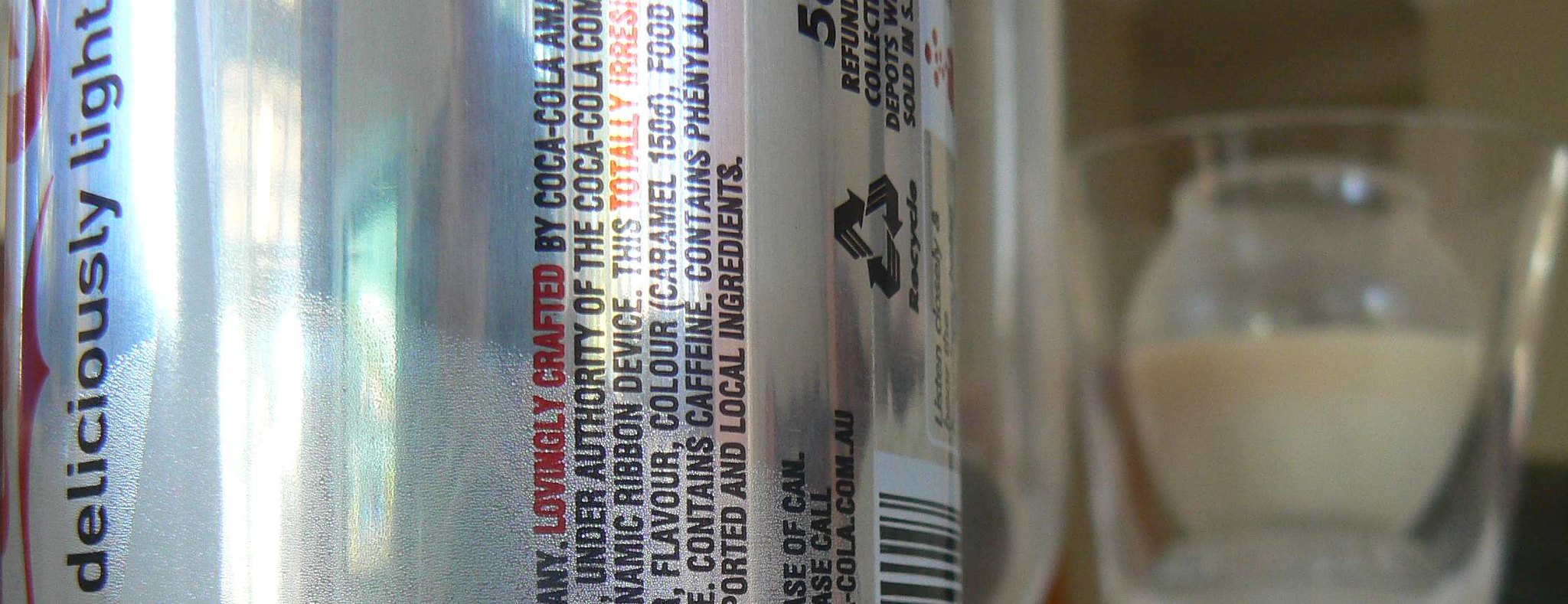This photo features a silver can of Coca-Cola positioned on the left side of the frame. Prominently displayed on the far left of the can is the iconic red Coca-Cola logo. Just below the logo, the phrase "Deliciously Light" is printed in black text. Further to the right on the can, there is a label with red text reading "Lovingly crafted," and underneath it in black text, "by Coca-Cola, under authority of the Coca-Cola Company." Additional details on the label include mentions of a ribbon device, flavor, color, caffeine, and local ingredients. Toward the bottom of the can, there is a rectangular recycling symbol. In the background of the image, a glass jar is visible with a smaller, round jar inside of it, which is half full with an unidentified white substance.